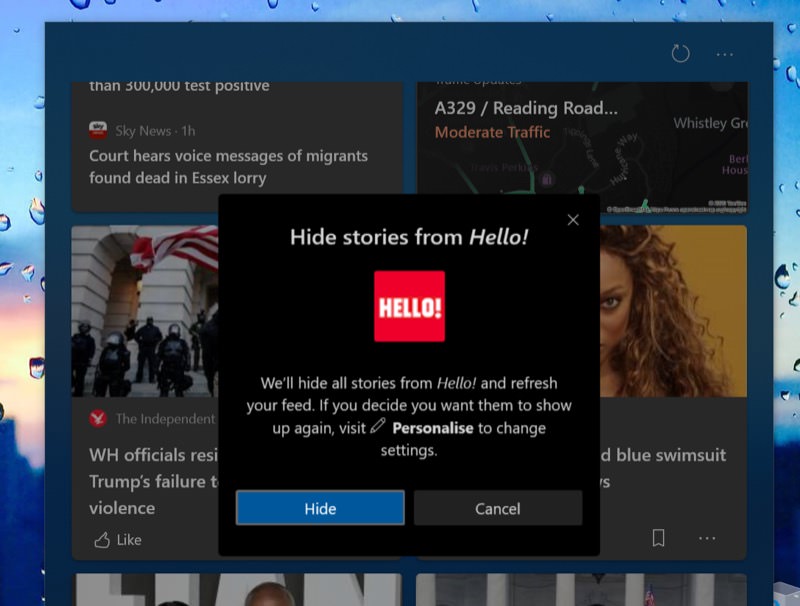This image features a computer screen displaying a navy blue window populated with several gray-toned tiles showcasing different news articles. Among the articles, one is marked from The Independent, another from Sky News, one appears to feature Tyra Banks, and another is categorized under traffic updates. The background of the main window is framed by the desktop wallpaper of the person's PC, which displays raindrops on a glass surface with a cityscape faintly visible. Overlaying the primary window is a jet-black pop-up window with white text. At the top of this pop-up, it reads "Hide stories from Hello" and below that displays the Hello logo, a red square with "hello" written in white. The pop-up continues to explain that all stories from Hello will be hidden and the feed refreshed, with the option to visit the "edit" or "pencil" icon to personalize settings if the user wishes to change them in the future.